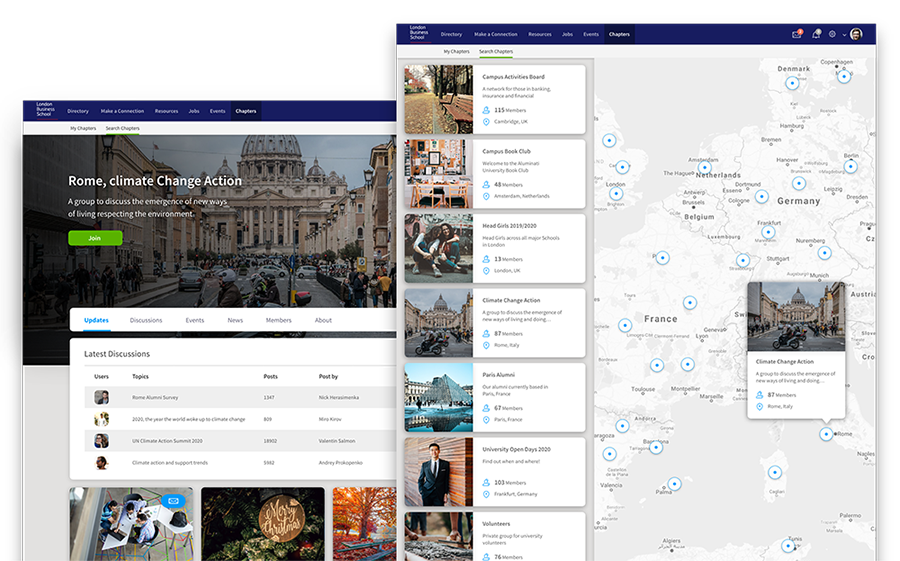The image showcases two overlapping screenshots of the London Business School's website, both identifiable by the dark blue menu bar and the logo at the top left corner. The right-hand screenshot overlaps the left-hand one, presenting a more vertical layout. This page prominently features a map of Europe highlighting regions such as France, Germany, Belgium, and the Netherlands, marked with blue circles to denote various locations. Adjacent to the map, a columned list with cover pictures categorizes different sections related to these locations.

At the top right of this vertical page's menu bar are several user icons: a mail icon with a red notification circle, a bell icon with a gray notification circle, an arrow dropdown icon, and a circular profile icon displaying a blurred image of a man.

The left-hand screenshot has a more horizontal orientation. It displays a wide cover picture of Rome, accompanied by the text "Rome Climate Change Action" and a green "Join" button. Below this, there are tabs for updates and website tools, along with a list of the latest discussions categorized by users and topics, followed by additional cover pictures. Despite the general blurriness of the screenshots, the consistent elements across both confirm they belong to the same website.